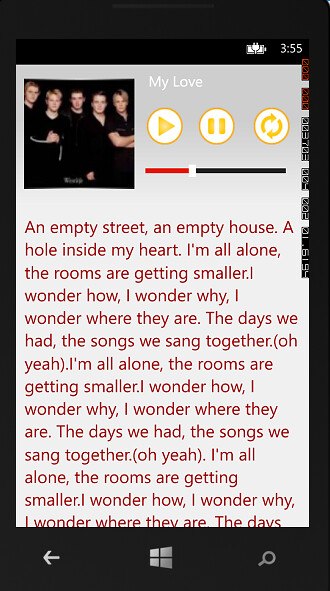This screenshot, taken from a phone at 3:55, features song lyrics displayed on a black and gray background. At the top left, there's a battery icon with a charging cord symbol. Below it, on a light blue section of the screen, there's an image of five boys in black attire, presumably the boy band singing the song. To the right of the image, "My Love" is displayed prominently, indicating the song title. Below this, there are playback controls, including play, pause, and refresh icons, next to a partially red and black progress bar. The lyrics shown include: "An empty street, an empty house, a hole inside my heart. I'm all alone, the rooms are getting smaller. I wonder how, I wonder why, I wonder where they are. The days we had, the songs we sang together, oh yeah." These lyrics repeat, cutting off midway through the phrase. At the very bottom of the screen, there's a navigation bar with an arrow pointing left, the Windows logo, four squares, and a magnifying glass icon on the right.